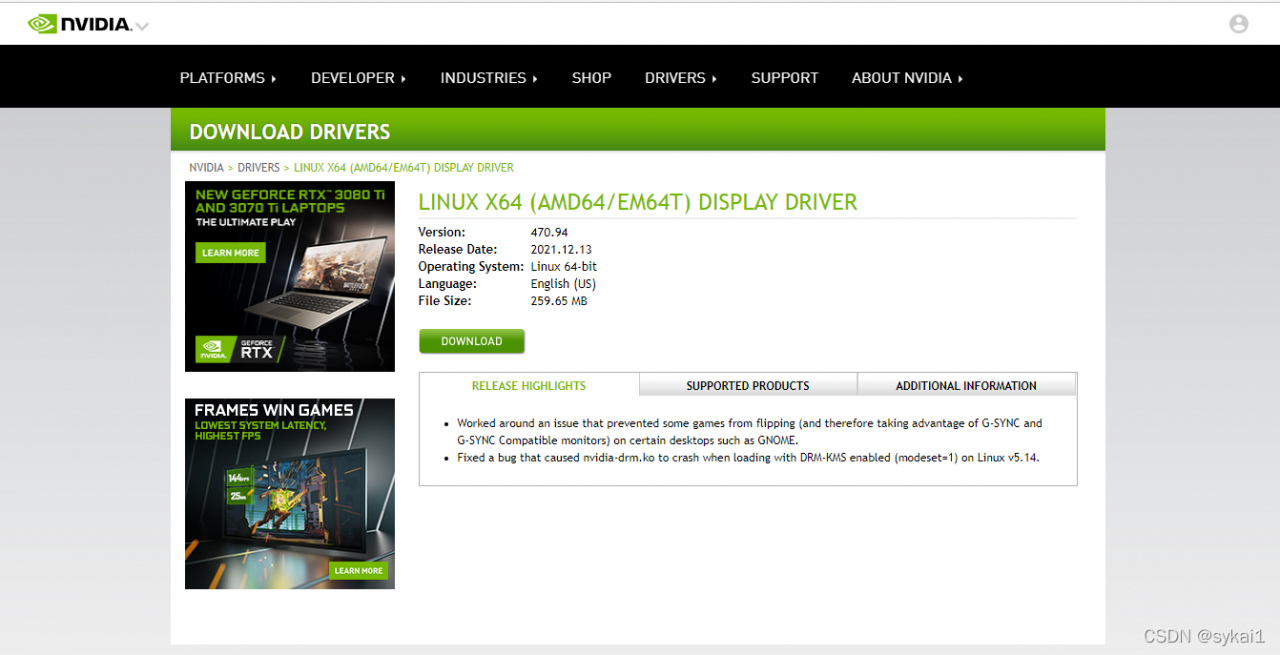The image is a detailed, colorful screenshot designed for a website's driver download section.

At the very top, there is a white banner featuring the NVIDIA logo in green, accompanied by "NVIDIA" written in black, positioned in the left-hand corner. Directly below this is a black navigation bar containing several clickable white tabs labeled: Platforms (with a right arrow), Developer, Industries, Shop, Drivers, Support, and About NVIDIA.

Beneath the navigation bar, the main content area starts with a prominent white section that includes a thin, bright green horizontal line at its top flanked by grey spaces. Centered within this white box is the text "Download Drivers," followed by the title "NVIDIA Drivers."

Further down, two images are displayed on the left side. One features an advertisement for the Neo GeForce RTX 380Ti and 370Ti, indicating these are laptop models with a "Learn More" prompt. The accompanying image shows a sleek laptop. Below this, there is another image depicting either a screen or a tablet, emphasizing gaming performance with the slogans "Frames Win Games" and "Lowest System Latency, Highest FPS."

To the right of these images is another informational section detailing a specific NVIDIA driver. It lists "Linux x64 (AMD 64/EM640) Display Driver," with the version 470.94, release date 2021-12-13. Additional details include the operating system compatibility (Linux 64-bit), language (English US), file size (259.6 megabytes), and a prominent "Download" button.

At the bottom of the image, there are sections for "Release Highlights," "Supported Products," and "Additional Information," providing more in-depth details about this driver release, though the specific content of these sections is not fully visible in the image.